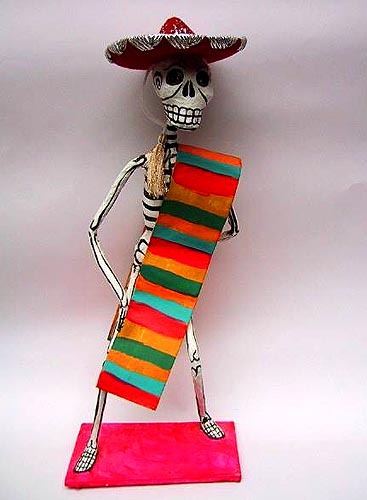The image is a color photograph featuring a small, handcrafted skeleton statue resembling Mexican folk art, most likely celebrating the Day of the Dead. The skeleton appears to be made out of clay and is intricately painted with a white body and black bones. The characteristically large, outlined teeth add to its festive appearance. It wears a predominantly red sombrero, trimmed with black and white details, and its black eye sockets give it a cheerful yet eerie expression. Draped over its shoulder is a colorful blanket, or serape, striped in vibrant shades of red, turquoise, yellow, and green, appropriately sized for the tiny skeleton. The statue’s left arm rests on its hip, while it stands on a pink, carpeted mat against a white backdrop, with no other visible surroundings. The overall scene suggests a celebration captured in a minimalist setting, emphasizing the colorful and cultural vibrancy of the figure.